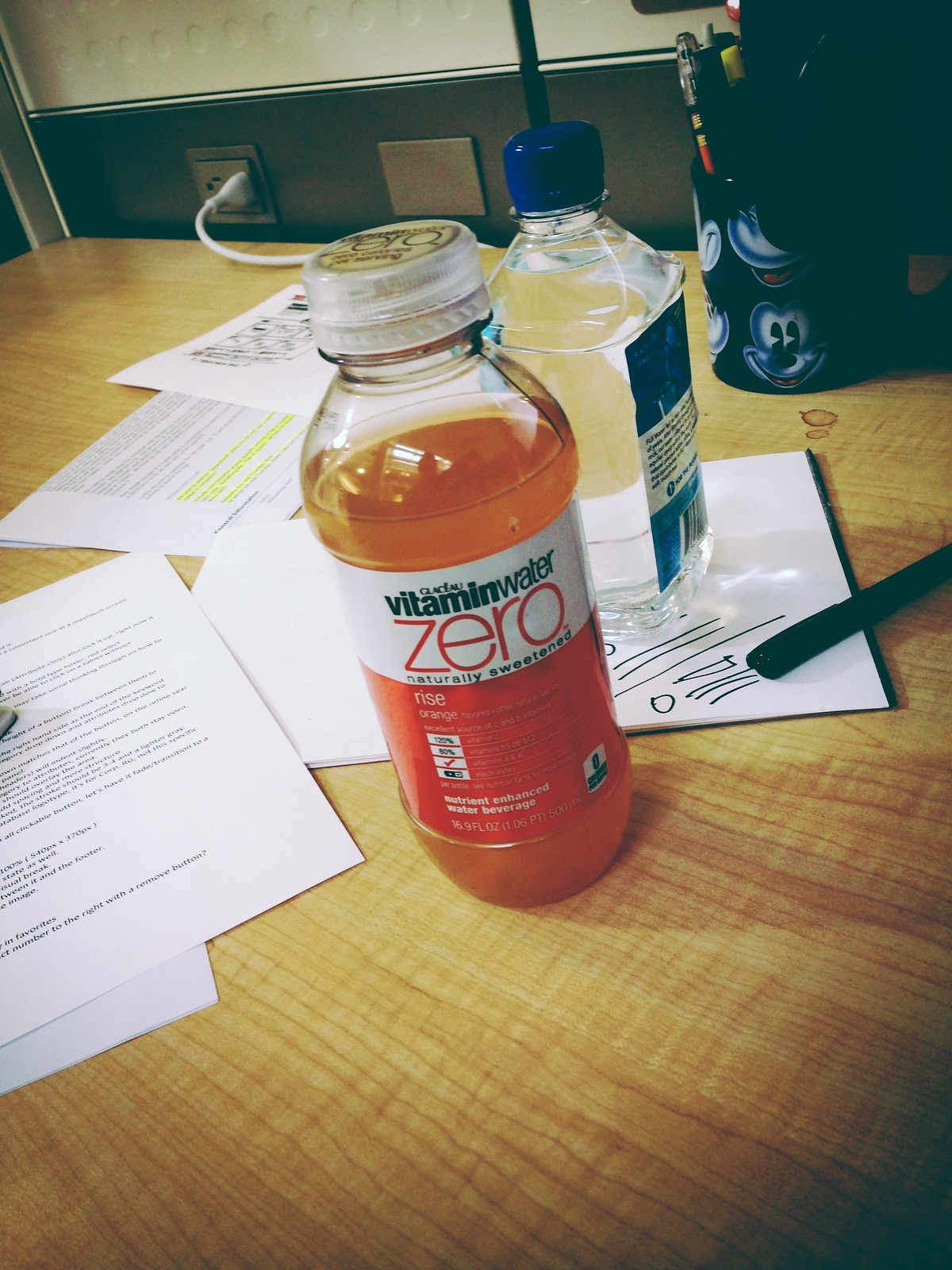This image captures a detailed view of an office desk setup. The desk itself is a light brown hue with a noticeable grain pattern in the composite wood surface. Scattered across the desk are various papers, some with highlighted sections and others without, giving a sense of an active workspace. 

Central to the image is a clear plastic bottle of Vitamin Water Zero, filled with an orange liquid up to four-fifths of its capacity. The bottle features a distinctive label: the top one-third is white with black text reading "vitamin water," red text saying "zero," and smaller black text stating "naturally sweet." The lower two-thirds of the label is a reddish-orange color. 

Behind this bottle stands another clear plastic bottle, identified as a Fiji water bottle, with a square shape and a blue cap. This bottle rests upon a white notepad. 

Additionally, a black Mickey Mouse coffee cup with white detailing is positioned at the upper right corner, holding several pens. An electrical outlet is visible in the background wall, with a single white cord plugged into it. The wall itself features a dark brown lower section topped with a lighter brown upper section, adding depth to the background.

Overall, the image conveys a busy and personalized workspace with distinct organizational elements and a variety of commonly used items.